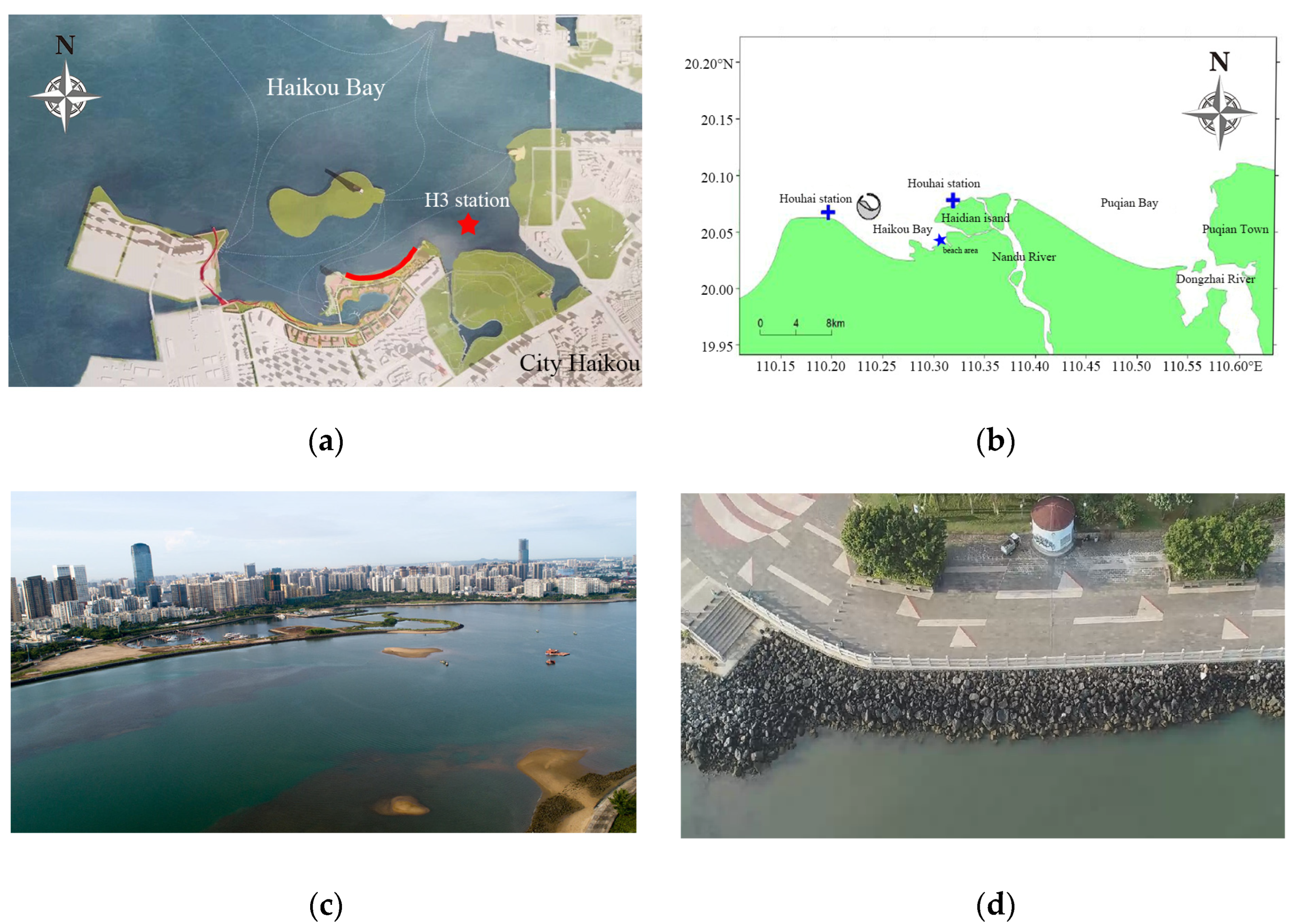This composite image consists of four labeled sections, A, B, C, and D, with two diagrams on the top and two photographs on the bottom, symmetrically arranged. 

**Diagram A (Top Left):** Labeled "Hayaku Bay" in white text at the top center, this colored map provides an overview of the area with a compass indicating north on the left side. The map displays various land pieces in white and green, surrounding a dark blue body of water. Noteworthy features include yellow lines on the center left, a deeper red line over a piece of land below a "figure-8" shaped landform in the water, the label "H3 Station" with a red star on the right, and "City Hokkaido" in the bottom right corner.

**Diagram B (Top Right):** This similar digital map includes several labels. On the left and bottom, it shows the location and features a compass marked with 'N' on the right side. A cross labeled "Hinobi Station" appears on the left, a star on a green land labeled "Hayaku Bay," and another cross labeled "Hinobi Station" to the right and upward. The "Dekuza River" is noted within a candy-cane shaped river, further marked "Kenku Town" and "Kenku Bay" to the right.

**Photograph C (Bottom Left):** This realistic cityscape photograph depicts tall buildings and a large river in the same area. The quality of the image highlights the urban area and its water features.

**Photograph D (Bottom Right):** Focused on the shoreline, this close-up image shows a road, bushes, greenery, and a small white building with a brown spire. The photograph includes visible black rocks and road markings, enhancing the detailed view of the shoreline infrastructure.

Together, these four images provide a comprehensive, multi-perspective view of the Hayaku Bay and surrounding areas, combining both aerial schematic representations and ground-level photographs.